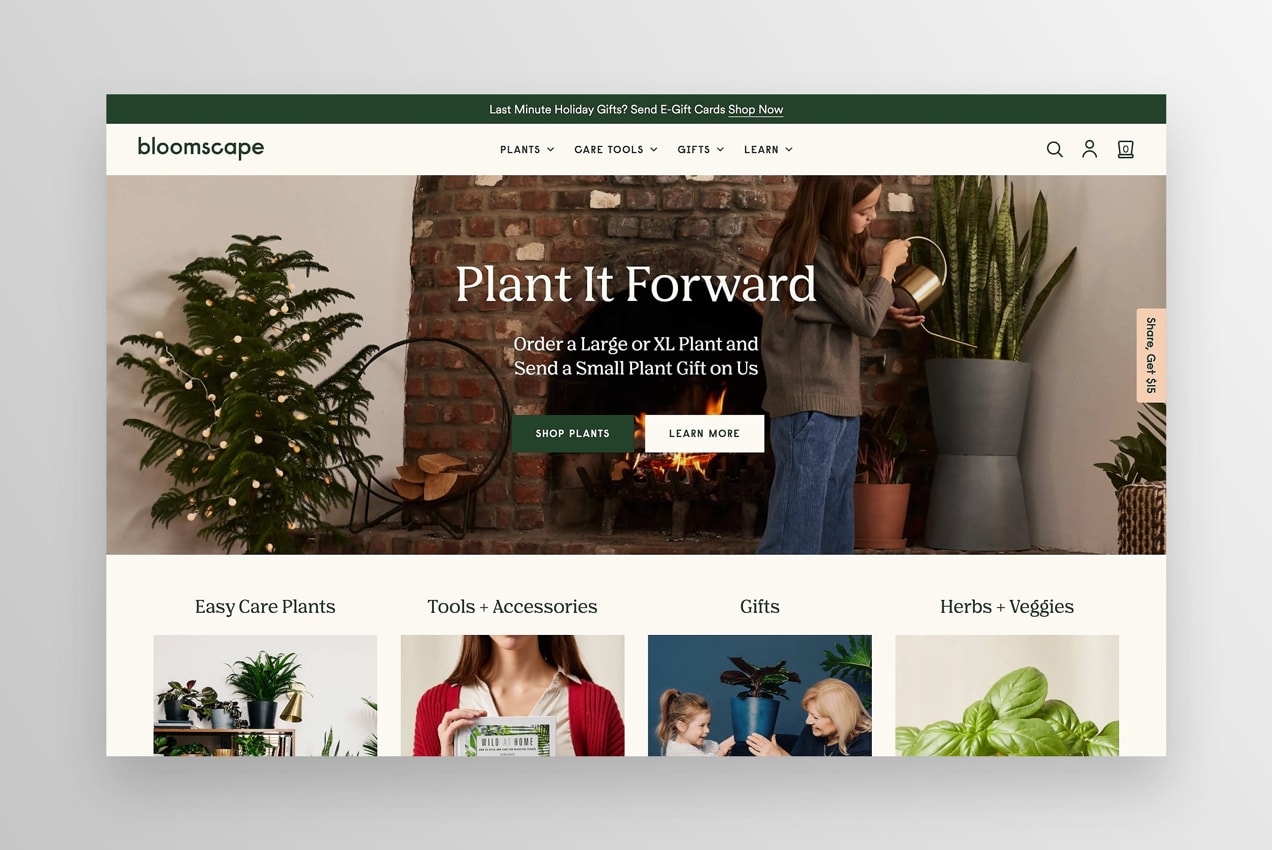The webpage titled "Plant It Forward" is a delightful haven for gardening enthusiasts and indoor plant lovers. At the very top, a dark sage green bar resembling the color of a pine tree sets a tranquil tone. Below this, the word "Bloomscape" is prominently displayed, leading into an organized layout featuring sections for plants, care tools, gifts, and learning resources.

The page showcases a serene image of a woman gently watering her snake plant. To her side stands a pine tree adorned with tiny white light bulbs, an enchanting touch. The season isn't clear, adding a timeless charm to the scene. 

Directly below, the "Easy Care Plants" section invites users to click and explore a variety of low-maintenance plants, ideal for busy individuals. Adjacent sections titled "Tools + Accessories," "Gifts," and "Herbs and Veggies" offer further exploration into plant care essentials and themed ideas. 

The page’s appeal is in its simplicity and beauty, making the world of plants accessible and inviting for all, especially those who appreciate easy-to-care-for options.